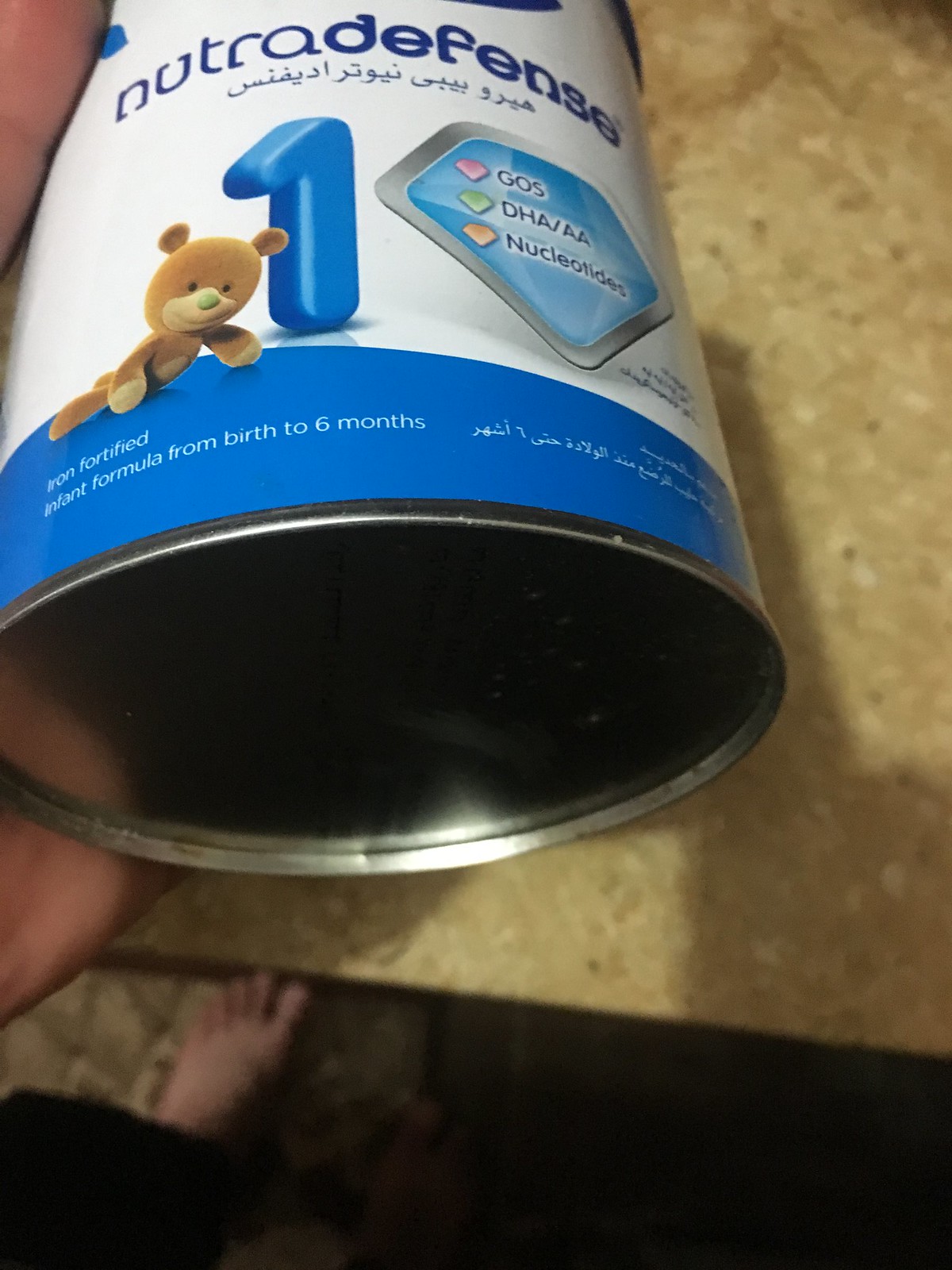In this eye-level photograph, the viewer looks down to see part of the photographer's leg and bare foot alongside a light brown counter with black specks. The photographer's hand holds a metal container with a blue and white label that reads "NutraDefense" in blue text. The can also features a 1 in blue beside an image of a brown teddy bear with a green nose. Below the main label, additional text in Arabic appears, along with a blue and gray diamond-shaped box containing the words "GOS DHA Nucleotides." At the bottom edge of the can, a blue stripe bears the inscription "Iron Fortified Infant Formula from birth to six months" in white letters. The inside of the can is lined with silver, and the intricate label design includes a silver diamond outline with a heart shape in red, green, and orange on a blue background.